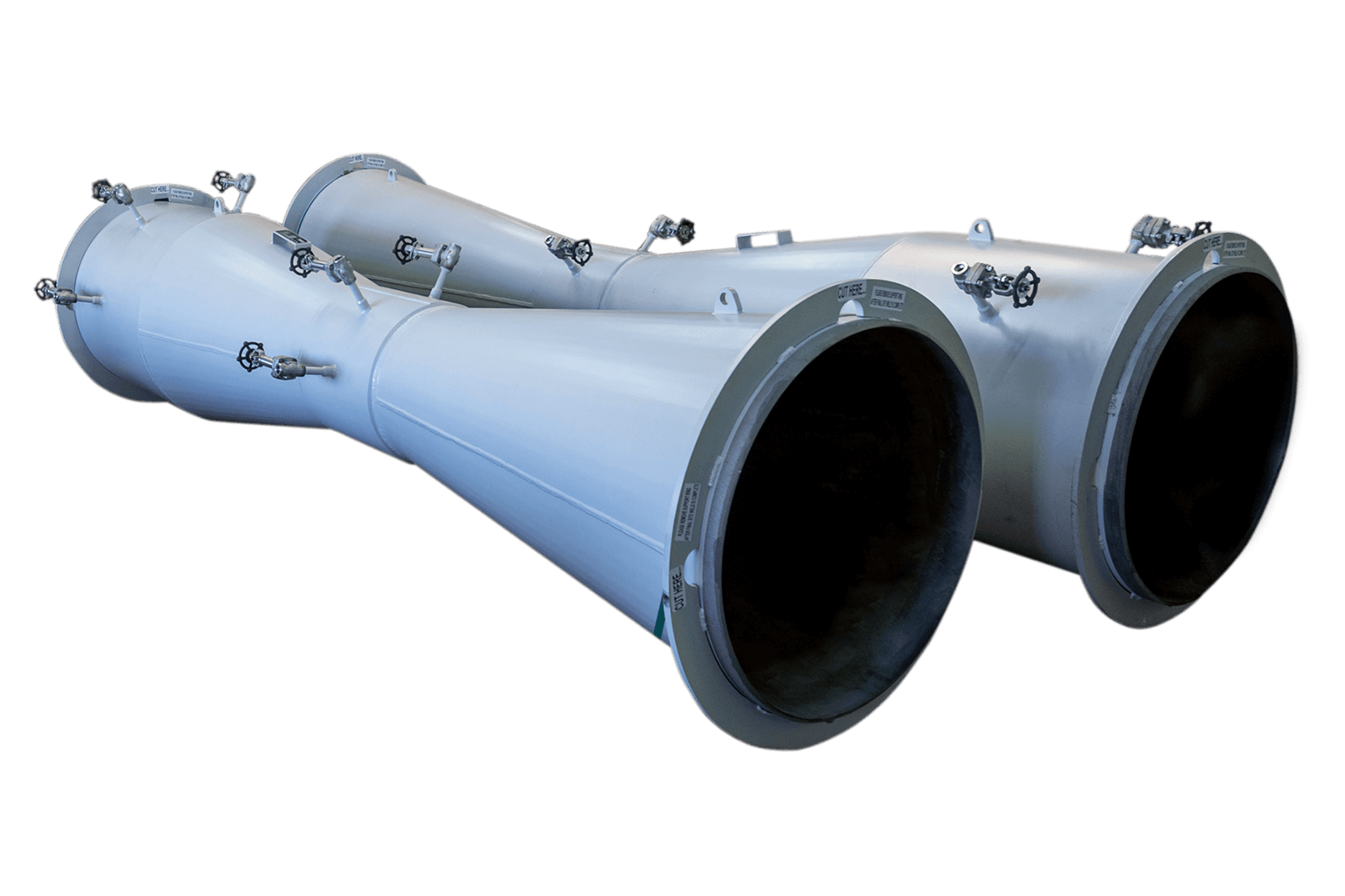The image showcases two large, light gray cylindrical objects lying side-by-side, resembling industrial equipment. These structures have wide, flanged bases that taper into smaller cylindrical tops. Each is equipped with numerous black faucet-like handles and metal gears, possibly for controlling the flow of a substance. The objects have several small pipes and turnwheels attached to them. Although they are hollow and feature open ends, they could serve as connecting pipes or some form of conduit. Despite their industrial appearance, their exact purpose is unclear, reminding viewers of oversized binoculars or torpedo tubes due to their significant size and symmetrical placement.